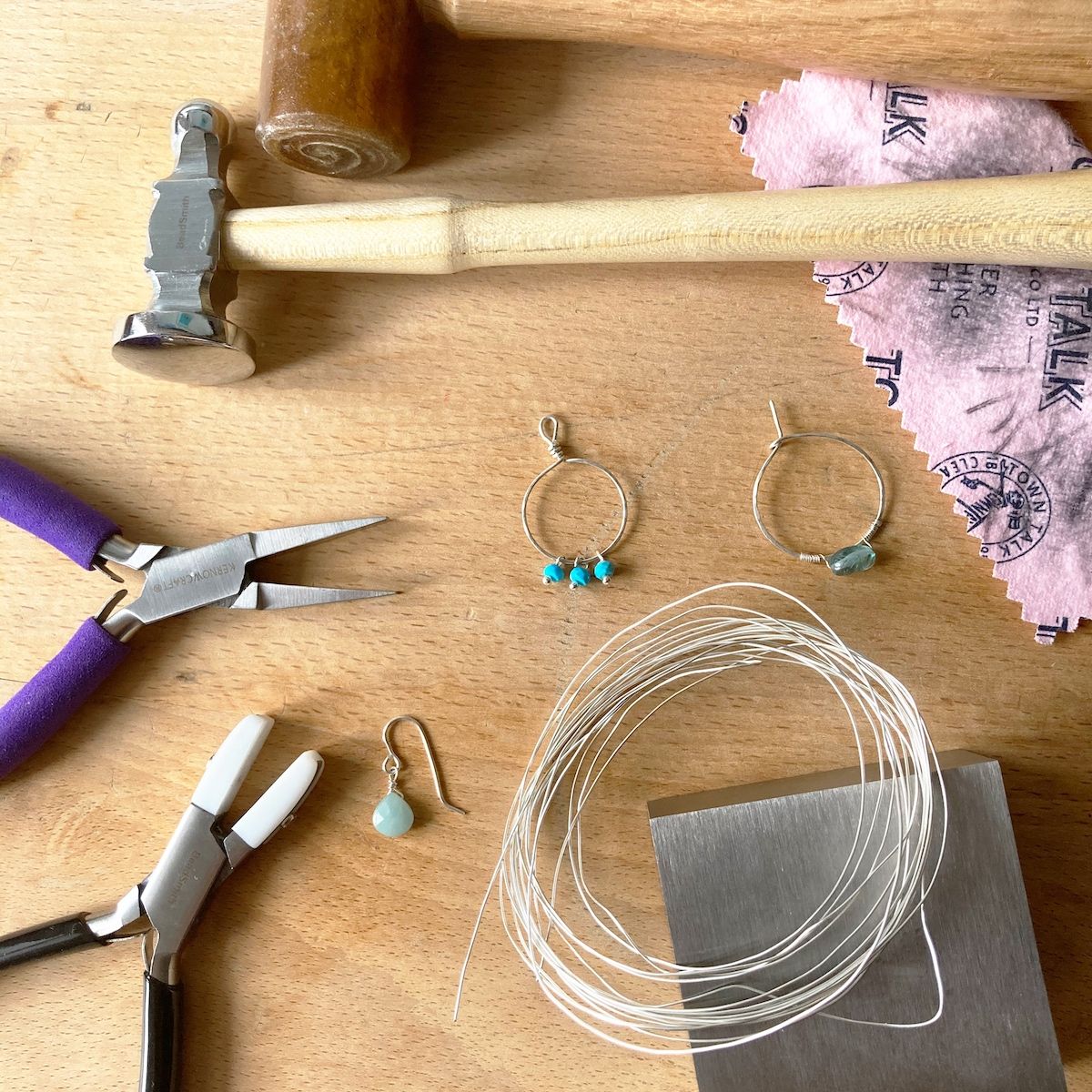The photograph depicts a light brown, wooden tabletop cluttered with a variety of tools and jewelry pieces. In the top section of the image, there is a hammer with an off-white handle and a gray metal head placed above a light pink cloth that has "Town Talk" emblazoned in black on it. Below the hammer's handle and slightly to the right rests two sets of hoop earrings adorned with light blue beads. Centered towards the middle right, a coiled piece of white string or wire is visible, possibly resting on a shiny metal cube.

In the bottom left corner of the table are two pairs of pliers: one with needle-nose tips and purple handles, and another pair with black handles lying just beneath it. Nearby, an earring embellished with a round, light blue, pearl-like stone is also noticeable, adding to the array of scattered items. The detailed arrangement captures a workspace that blends tool usage with jewelry crafting, marked by a mix of functional and decorative items spread across the wooden surface.